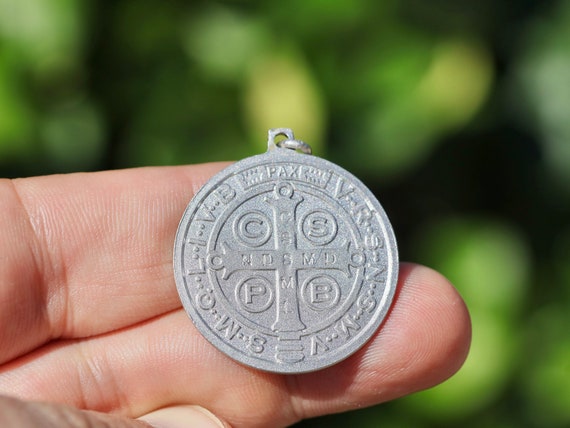In this detailed close-up photograph, a person's white index and middle fingers are holding a circular silver necklace pendant, distinctly vintage in appearance. The necklace pendant, detailed with a cross at its center, features small hoops or circles at each end of the cross, each inscribed with the letters C, S, P, and B. Additional inscriptions on the cross include the letters NDSMD and CSSMI. Surrounding the cross, the pendant is further engraved with letters reading SMOLIVB and VRSNSMV. Near the top, the word "PAX" is inscribed, and above it is a small metal clasp, designed to attach to a chain but currently unattached. The blurred, green background, likely foliage, frames the pendant's intricate details, highlighting its possible origin from a religious ceremony, with text that might be Latin. The thumb of the person holding the pendant is also visible, adding a subtle human element to the intricate, historical piece.